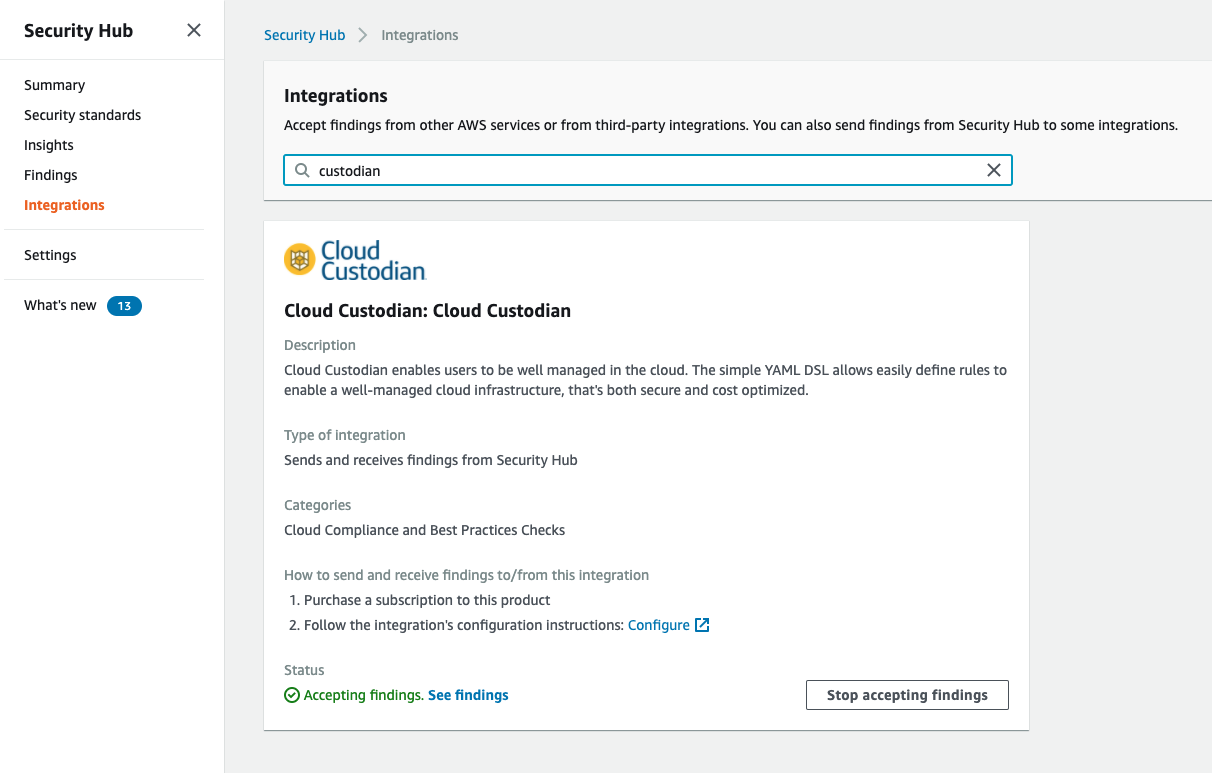In the image, the user is viewing the Security Hub page within the Amazon Web Services (AWS) interface. The layout includes a navigation pane on the left side, listing sections like "Summary," "Security Standards," "Insights," "Findings," "Integrations," "Settings," and "What's New." A notification bubble displaying the number '13' is next to the "What's New" section, indicating new updates or alerts.

The main pane focuses on the "Integrations" section. The description explains that in this section, users can accept findings from other AWS services or third-party integrations, and can also send findings from Security Hub to these integrations. Below this explanatory text, there is a search bar where the user has typed in "custodian."

The search result highlights an integration called "Cloud Custodian," which comes with a small logo. This integration helps users maintain a well-managed cloud environment by defining rules for infrastructure management. The purpose of this integration appears to be enhancing the user's ability to manage and secure their cloud setup through AWS by incorporating functionalities from other software applications. The user seems to be in the process of adding this Cloud Custodian integration to their AWS services.